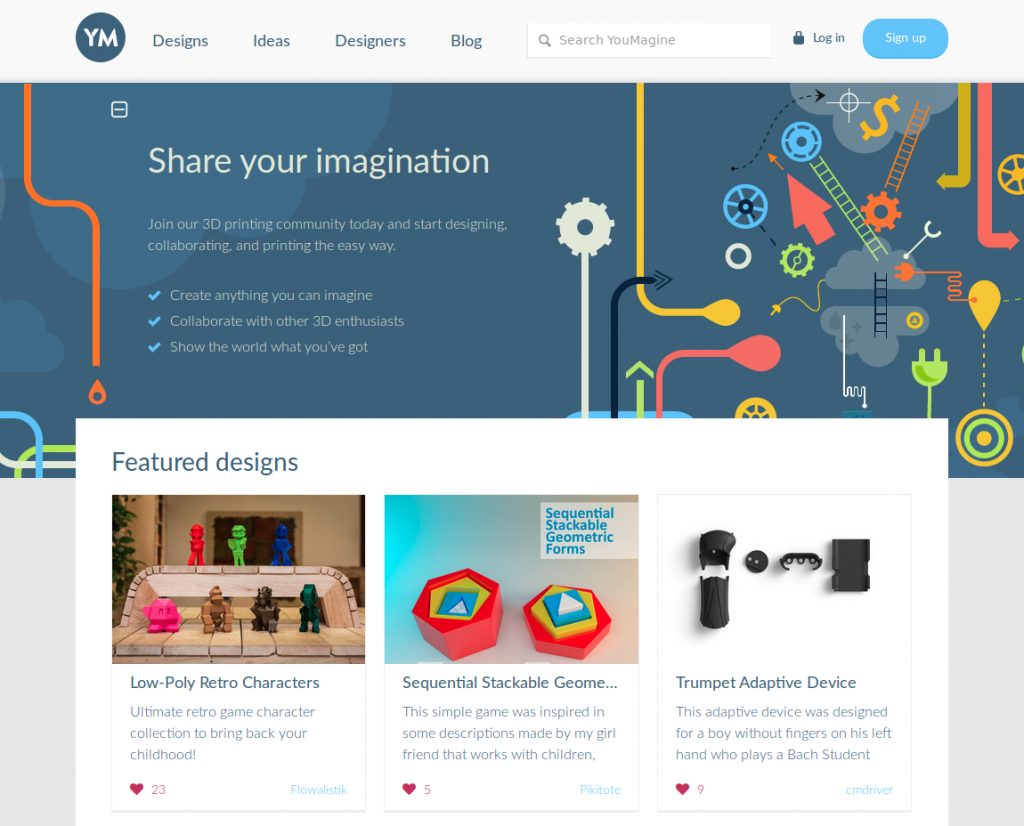This landscape-oriented screen capture appears to be from a laptop or desktop computer, showcasing a web page from a site named "You Imagine." The top portion of the image features a standard rectangular header with a light gray background. In the upper left corner, there is a circular dark blue logo with white capital letters "Y" and "M," representing "You Imagine." To the right of the logo, there are navigation options labeled "Designs," "Ideas," "Designers," and "Blog." Following these, there is a standard search bar with a magnifying glass icon and the placeholder text "Search." To the right of the search bar, there is a lock icon followed by the words "Log in," and a stretched blue oval button with the text "Sign up" in white.

The main content below the header is divided into two distinct sections. The top section has a dark blue background adorned with various multicolored lines and shapes, including orange, yellow, and white lines. On the left side, white text reads "Share your imagination," followed by a smaller-font checkmark list with light blue check marks:

1. Create anything you can imagine.
2. Collaborate with other 3D enthusiasts.
3. Show the world what you've got.

The right side of this section features an array of colorful graphics, including bent lines, arrows, a white gear shape, a green plug icon, a yellow dollar sign, gray clouds, and two angled ladders—one bright green and the other orange—along with a thick orange arrowhead.

The bottom section features a light gray background with a central white rectangle, slightly smaller than the section itself. At the top left of the white rectangle, the text "Feature Designs" is displayed. Below this are three images representing featured designs:

1. The left image depicts plastic figurines labeled "Low Poly Retro Characters," accompanied by three lines of descriptive text and a red heart symbol indicating 23 likes.
2. The middle image shows sequential stackable geometric forms with hexagon shapes in orange, yellow, and blue, labeled "Sequential Stackable Geometric Forms." This image also has three lines of descriptive text, ending with an ellipsis due to length, and a red heart symbol indicating 5 likes.
3. The right image features black plastic pieces labeled "Trumpet Adaptive Device," with three lines of descriptive text and a red heart symbol indicating 9 likes.

This detailed layout highlights the interactive and creative focus of the "You Imagine" website, catering to 3D design enthusiasts.